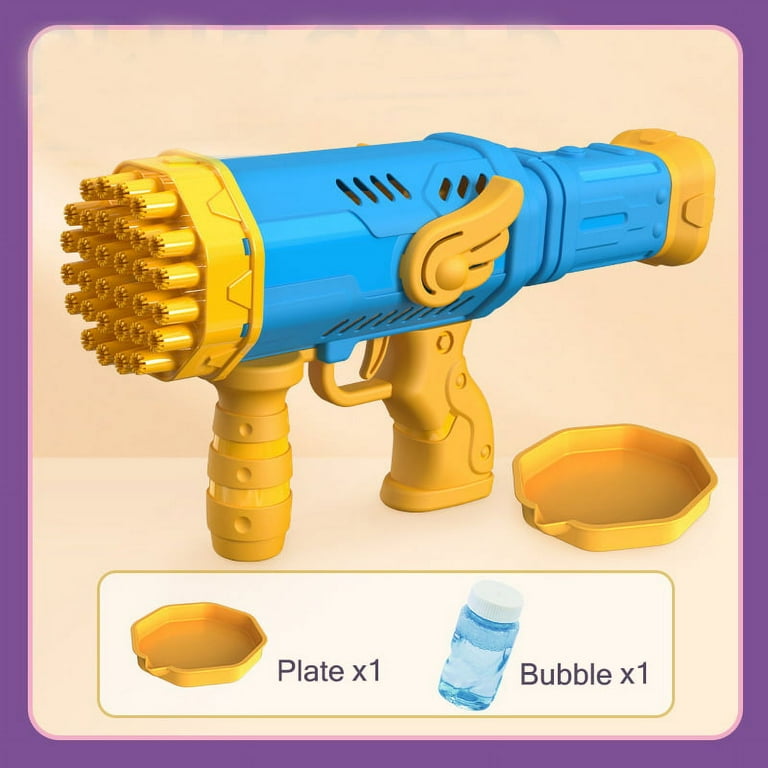This image showcases a child's elaborate bubble-blowing gun set against a pale yellow background, framed by a purple border. The bubble gun features a light blue body with yellow accents, including the edges, handle, and trigger. The forefront of the device boasts a series of multiple bubble outputs, designed to release approximately 24 bubbles simultaneously. The gun's detailed structure includes two handles at the base and an extended yellow piece for stability. Additionally, the set includes a circular, yellow bubble plate with an integrated spout for easy bubble pouring and a bottle of bubbles, both of which are displayed in a white pull-out box at the bottom of the image.